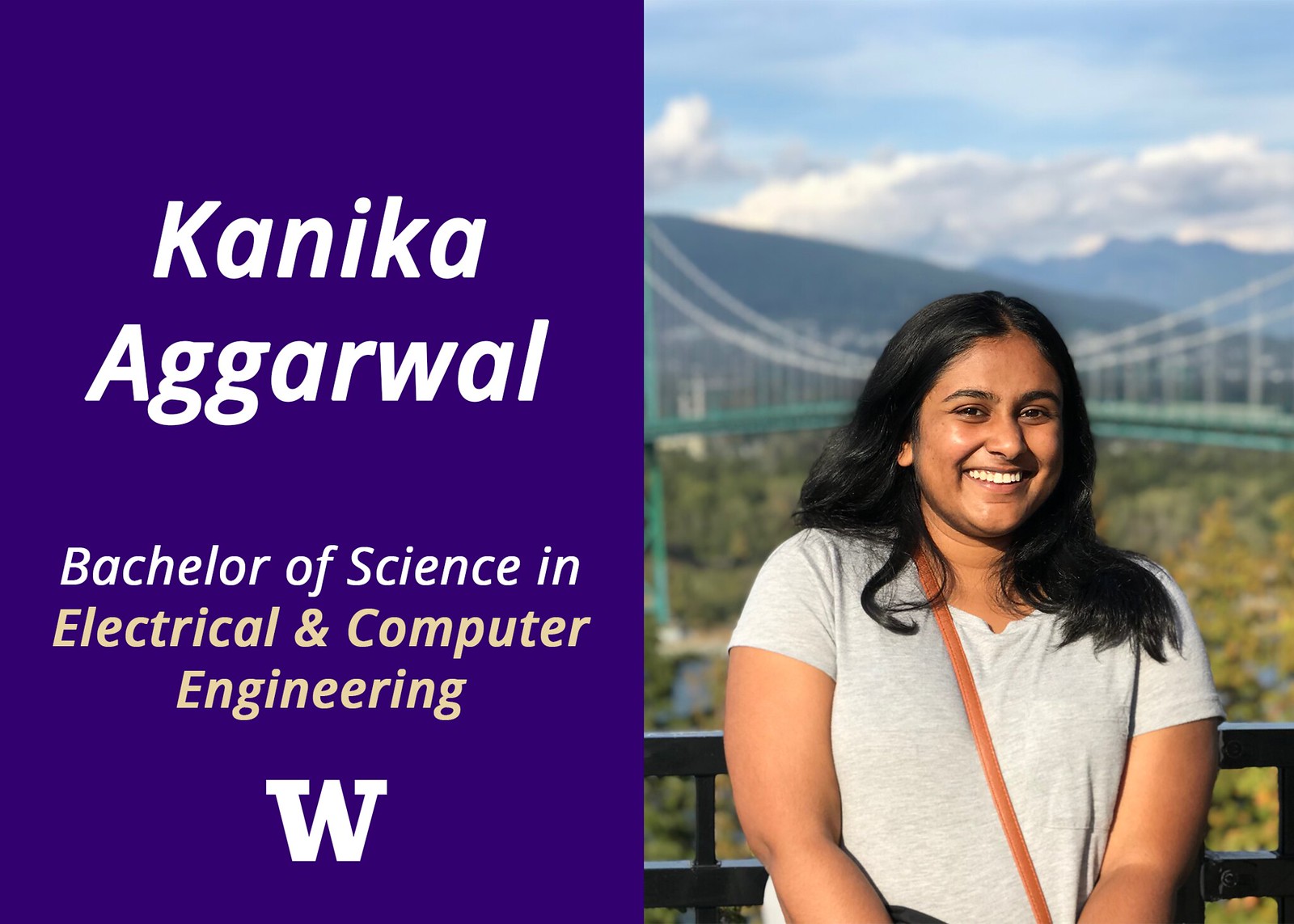This introductory banner, likely for a website or a graduation announcement, features a professional photograph of a young Indian woman named Kanika Agarwal. She appears to be in her late teens or early 20s, with long, dark black hair, and she is smiling warmly at the camera. Kanika is wearing a white T-shirt and has a light brown strap of a purse slung across her torso. The background showcases a scenic view with a teal suspension bridge, forested areas, and mountains under a blue sky with clouds, all slightly blurred due to the depth of field used in the photograph.

On the left side of the banner is a solid blue section displaying her name, "Kanika Agarwal," in large white text, followed by "Bachelor of Science in Electrical and Computer Engineering." At the bottom of this text section is a large white "W" logo, indicating a campus affiliation. The combination of Kanika’s bright smile and the picturesque setting creates an inviting and professional representation of a recent graduate.